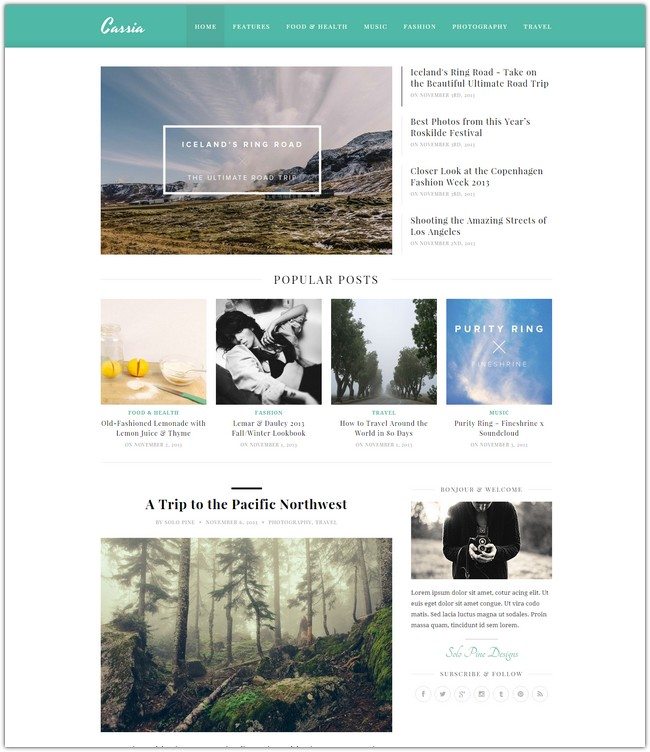Here is the cleaned-up and detailed caption for the screenshot of the webpage:

---

This screenshot showcases a webpage titled "Kaseya," identifiable by the teal-colored top header. The website's name, "Kaseya," is prominently displayed on the left side of the header. Adjacent to the site name, there is a menu bar with the following navigational options: Home, Features, Food and Health, Music, Fashion, Photography, and Travel.

Below the header, the rest of the webpage features a white background, serving as an articles page. This section includes images and titles of various articles. The first prominent image is of Iceland's Ring Road, providing a picturesque view of Iceland's rugged mountain landscape. To the right of this image, there are four rows of article titles:
1. "Iceland's Ring Road: Take a Beautiful Ultimate Road Trip"
2. "Best Photos from the Year's Rock Slide Festival"
3. "Closer Look at Copenhagen Fashion Week 2013"
4. "Shooting the Amazing Streets of Los Angeles"

Directly below these articles is a section titled "Popular Posts," centered within the webpage. It features four images in a row:
1. An image for the "Food and Health" category
2. A black and white photograph of a model in a bikini and bolero jacket, representing "Fashion"
3. A "Travel" image showing a straight road flanked by trees disappearing into the fog
4. An album cover for Purity Ring's "Einstein," symbolizing "Music"

Further down, there is an article titled "A Trip to the Pacific Northwest," accompanied by a photograph of a foggy forest with dense trees and moss-covered ground. Adjacent to this, on the right side, is a smaller box titled "Bonjour and Welcome," featuring a vintage black and white photograph of a man holding an old-fashioned camera, with some introductory text below.

At the very bottom of the page, there's a "Subscribe and Follow" section with a row of social media icons, including Facebook, Twitter, Google+, Instagram, Tumblr, and an RSS feed icon.

---